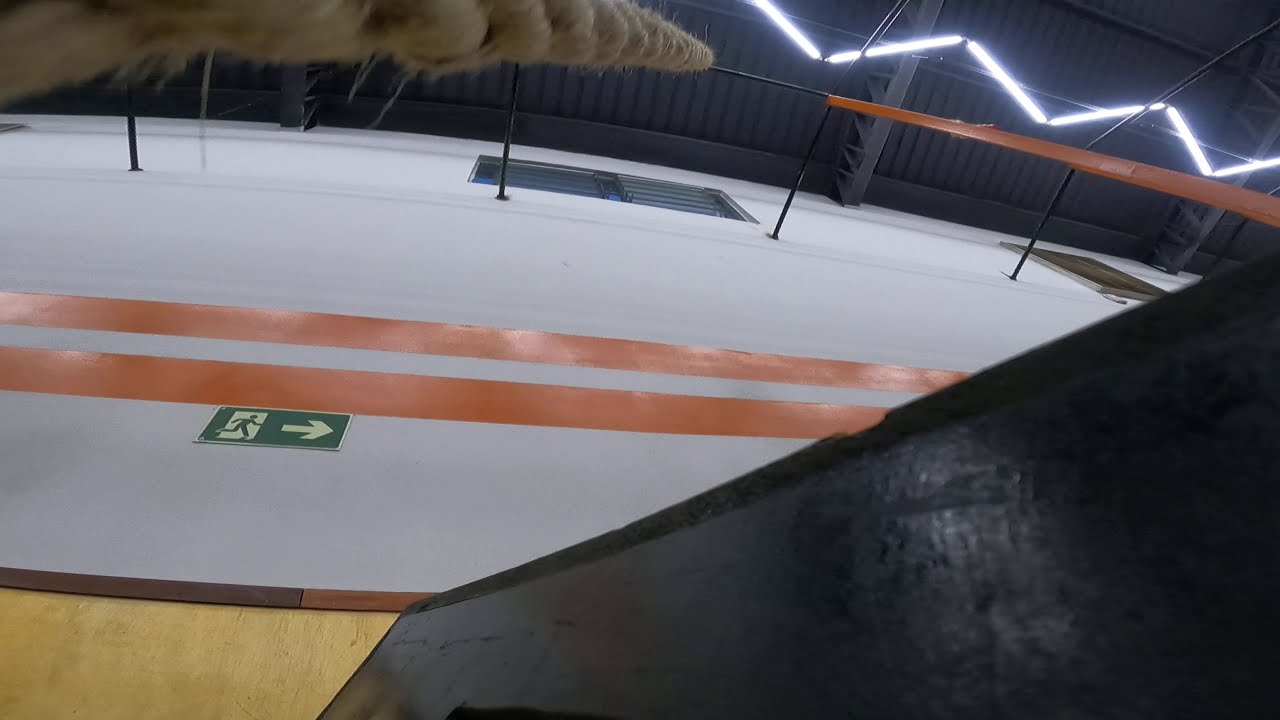This color photograph, taken from a low angle, captures the interior of a warehouse-like building with a black, corrugated metal ceiling and fluorescent lights arranged in a zigzag pattern. The focal point is a white wall adorned with two horizontal orange lines extending across its width. Below these lines, a green safety sign featuring a white arrow pointing to the right and a running pedestrian figure can be seen. The bottom left corner of the image reveals a light wooden baseboard, while the bottom right is dominated by a large, black, boxy shape that appears close to the camera. A thick, light brown rope hangs prominently from black support beams near the ceiling, descending towards the viewer from the top left of the frame. The scene's vivid details and realistic representation offer a comprehensive glimpse into the industrial interior.